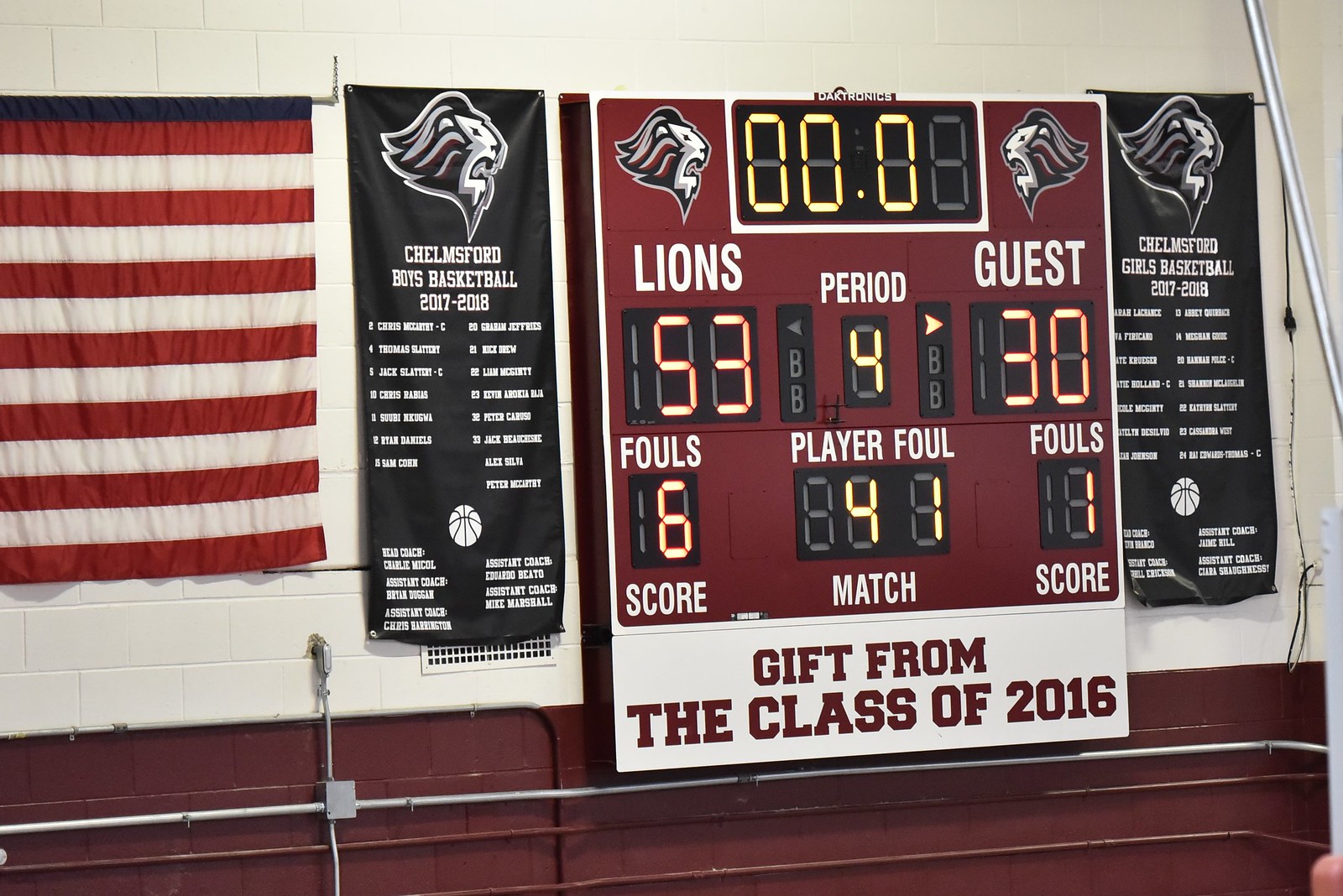A detailed caption for the described image:

The image captures the scoreboard in Chelmsford High School's gymnasium, displaying the final score of a basketball game where the Chelmsford Lions triumphed over their opponents with a decisive 53 to 30 victory. The scoreboard indicates that the game consisted of four periods, with the Lions accruing six fouls compared to the guests’ one. The scoreboard itself is a modern installation, a generous gift from the Class of 2016. Surrounding the scoreboard are banners celebrating the Chelmsford Boys and Girls Basketball rosters from the 2017-2018 seasons, highlighting the players and coaches. To the left of the scoreboard, an American flag is prominently displayed, adding a patriotic touch to the gym's decor. The overall scene reflects the pride and spirit of the Chelmsford High School basketball community.